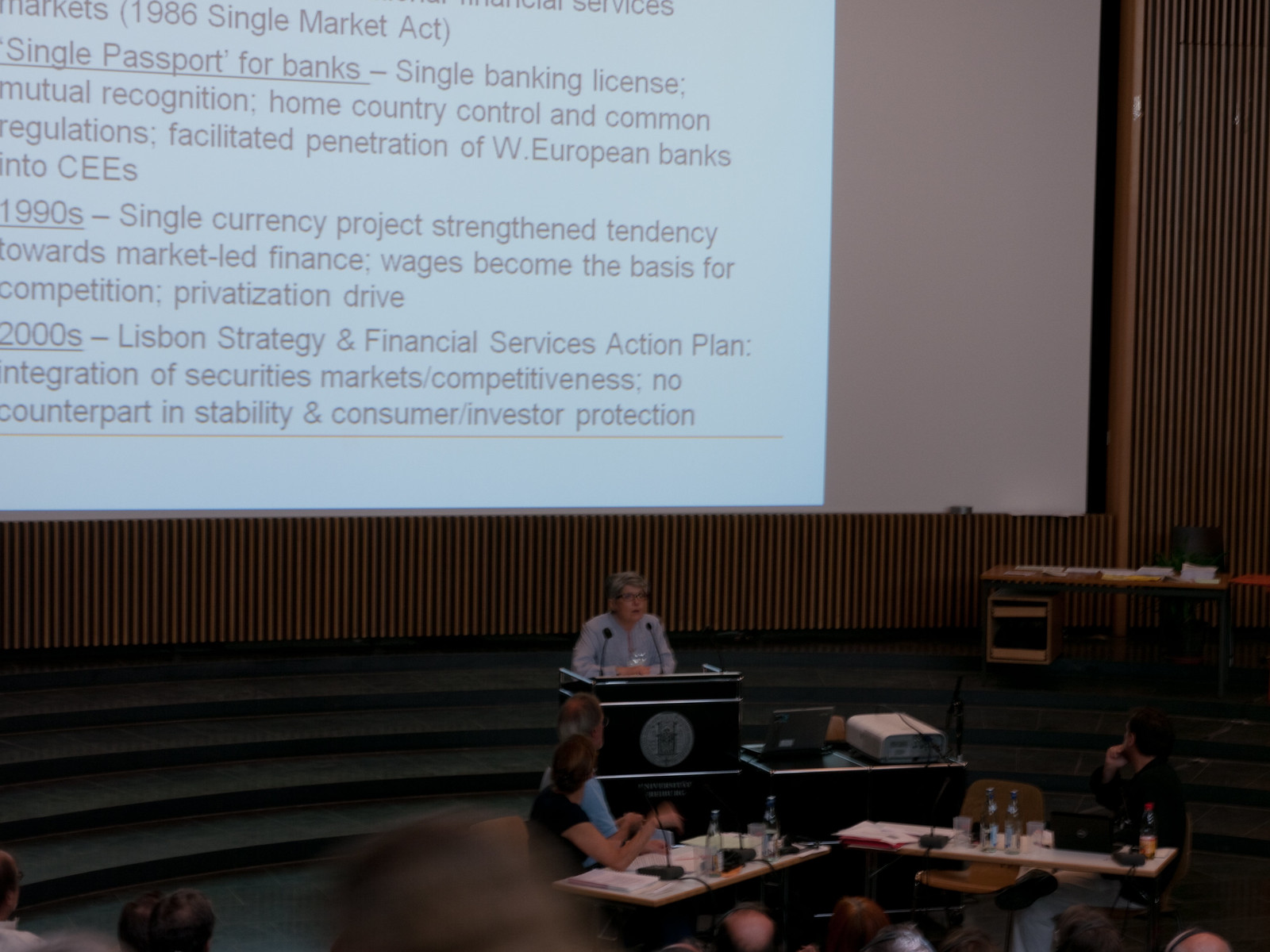The image depicts a middle-aged woman with short gray and black hair, wearing glasses and a gray blazer, standing at a black podium with two microphones. She is situated at the bottom center of the image in a dimly-lit auditorium, giving a lecture possibly to students. The audience, comprising mostly heads visible just above the bottom edge of the image, sits at tables facing her. Immediately in front of the podium, three attendees are facing back towards her, engaged in the lecture.

In the background, a large presentation is projected onto a whiteboard, with the text partially cropped. Legible portions detail topics such as the Markets 1986 Single Market Act, the 1990s single currency project, and the 2000s Lisbon Strategy and Financial Services Action Plan. Highlighted sections mention single passports for banks, mutual recognition, home country control, market-led finance, competitiveness, and consumer investor protection. The projection setup is flanked by vertical wooden panels and a set of dark stairs leading down to the speaker, adding structural and visual context to the scene.